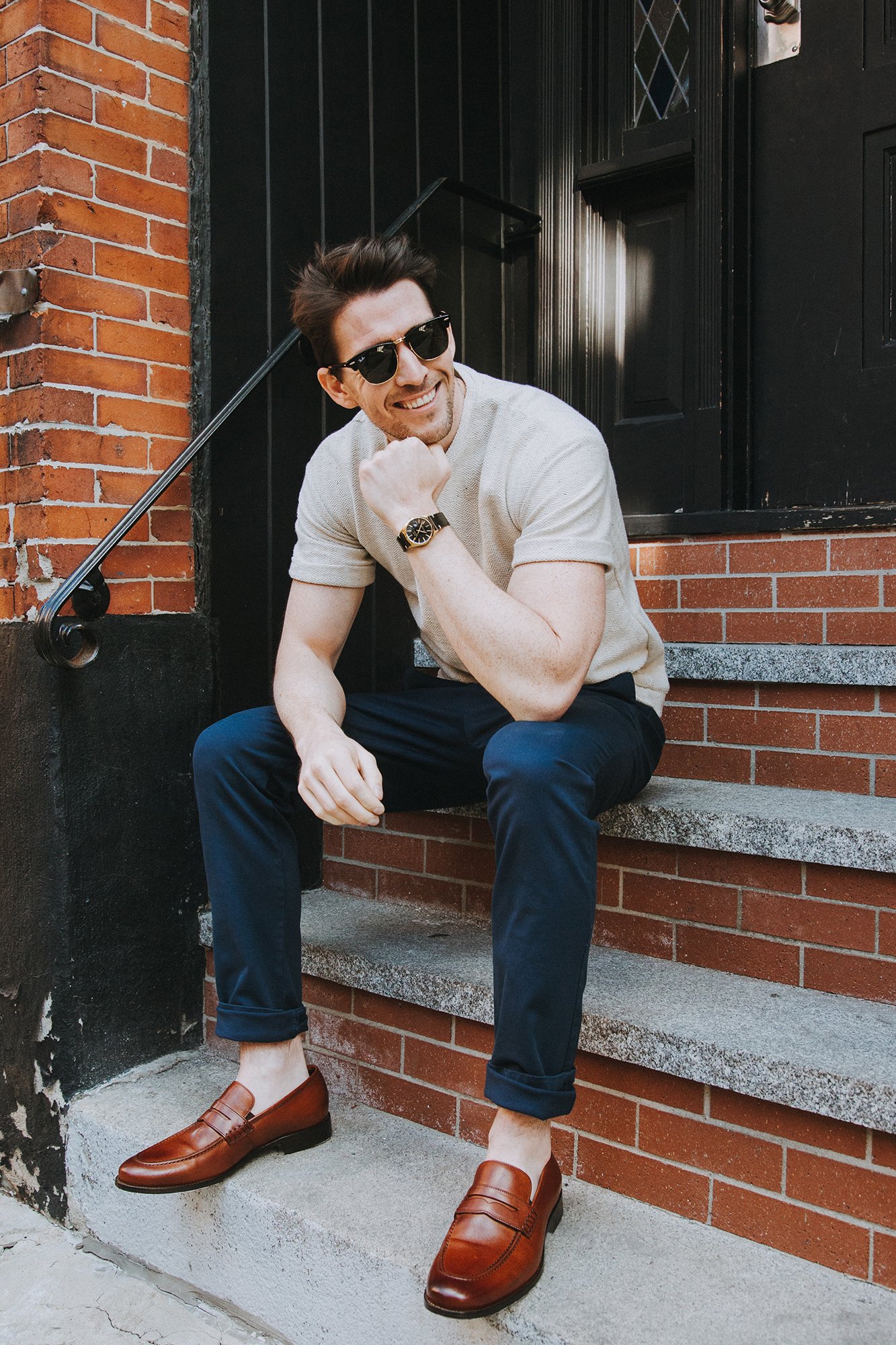In the photograph, a well-muscled young man is seated on the steps of a brownstone building, likely an apartment. He exudes a model-like presence, suggesting he is posing for the picture, given his confident demeanor and engaging posture. The man, who has long black hair and bears a slight resemblance to Tom Cruise, is dressed sharply in a beige t-shirt and blue pants, paired with brown penny loafers without socks. His stylish look is complemented by sunglasses and a watch. The scene captures him sitting with his arm resting on his knee, his fist under his chin, and a broad smile on his face, as he gazes to the left. The brick steps beneath him culminate in a gray concrete top, against the backdrop of a black door and the building’s brick façade. To the side, a glimpse of the gray sidewalk adds context to this detailed urban setting.